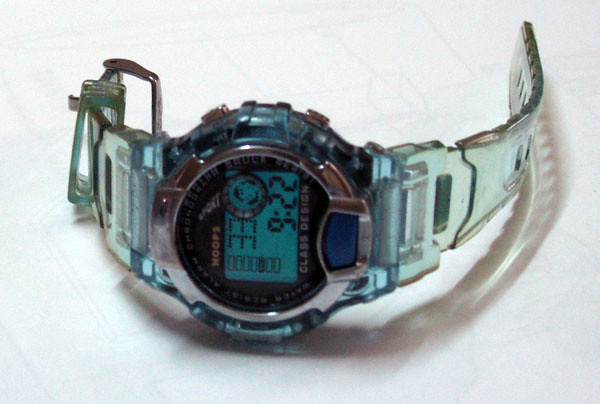Close-up image of a transparent digital sports watch placed on a subtly patterned white surface. The white background features faint geometric shapes, adding a touch of detail to the composition. The watch has a clear, round casing, within which the LED display is illuminated. The display shows multiple pieces of information: the top reads "Hoops," followed by "Sport." The time displayed is 9:22. Additionally, the words "Class Design" are visible, while the remaining text on the watch face is too small to decipher. The image focuses solely on the watch without any additional text or descriptive elements.